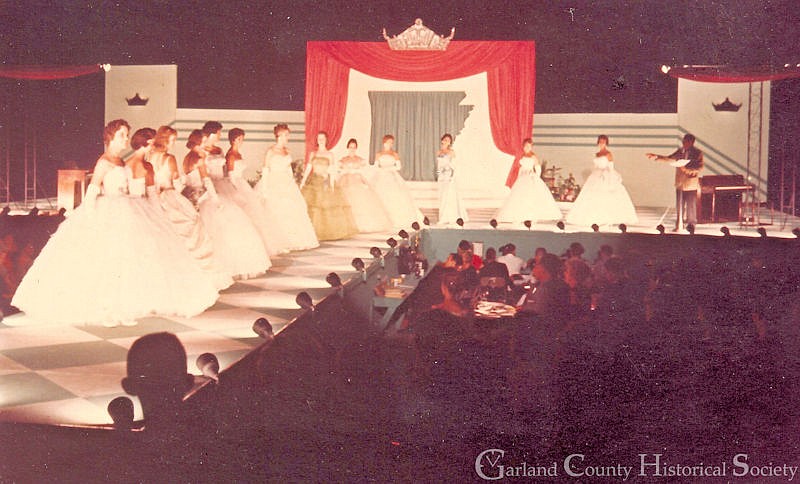The photograph, likely from the mid-20th century, showcases an elegant scene on the stage of an event organized by the Garland County Historical Society, as indicated by the label in the bottom right corner. The stage, shaped with a right-angle runway reminiscent of a fashion show, is populated by women dressed in extravagant white gowns, resembling wedding dresses. These women are adorned with long white gloves, and their hair is meticulously styled. Bright spotlights illuminate the entire stage, enhancing the refined atmosphere. Complementing the grandeur of the scene, crowns are displayed on archways at both sides of the stage, accompanied by a red curtain backdrop. A man in a suit stands near a piano in the right corner, seemingly directing the women. The audience, seated at tables, attentively watches the display, adding to the formal ambiance of the event.